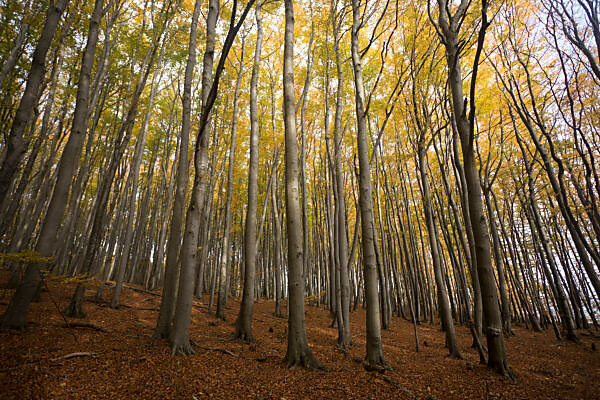This detailed photograph captures a serene forested hillside with an emphasis on tall, thin-trunked deciduous trees resembling aspens. Their trunks are uniformly brown and they stand at approximately 50 feet in height, spaced somewhat equidistantly, suggesting a possible landscaped arrangement. The canopy showcases a mixture of vibrant green and yellow leaves, through which diffused sunlight filters, illuminating the scene. The forest floor is covered with a soft golden-brown layer of dirt, dry leaves, and brush, giving it a mulch-like appearance. Above, patches of the partly cloudy sky can be glimpsed, predominantly blue and white, providing a gentle backdrop to the natural tableau. No people, animals, or vehicles disrupt the peaceful ambiance of this woodland setting.